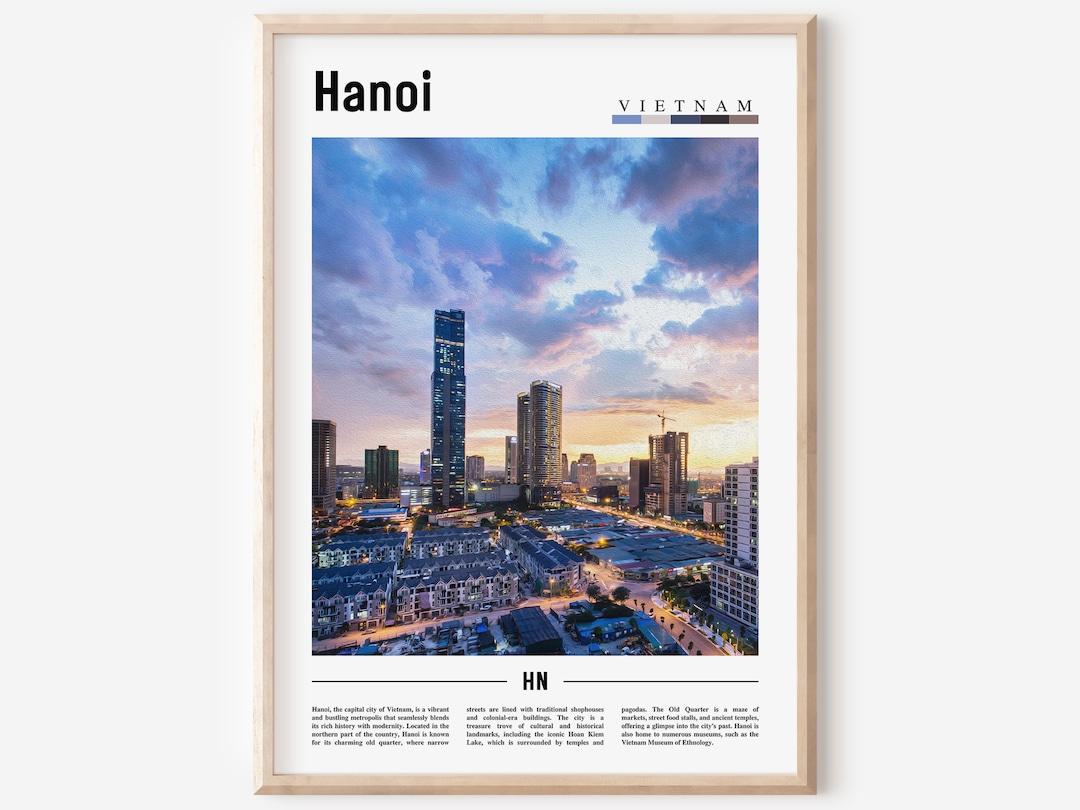On a pristine white surface sits a beige rectangular picture frame. Within the frame is a predominantly white image with a border comprising blue, white, black, and gray hues. The top left corner of the image bears the word "Hanoi" in black text, and adjacent to it, also in black, is "Vietnam." The central focus of the framed picture is a scene from Hanoi, the capital city of Vietnam. The city's skyline is captured under a sky adorned with clouds, possibly during sunrise or sunset. Tall skyscrapers dominate the landscape, providing a sense of the city's modernity. Green hues hint at the presence of the sun. At the bottom of the image, a caption reads: "Hanoi, the capital city of Vietnam. It's a vibrant and bustling metropolis that seamlessly blends its rich history with modernity."